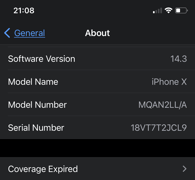In the screenshot, the time is displayed in the top left corner, reading "21:08" in white text. The screen appears to be set in dark mode, indicated by the black background and consistent use of white font throughout the image. At the top center, the title "About" is prominently displayed. To the left of the title, a blue hyperlink labeled "General" is visible, accompanied by a back arrow symbolizing a back key.

Below this header, detailed information about a cell phone is listed. The software version is "14.3," the model name is "iPhone X," and the model number is "MQAN2LL/A." Additionally, the serial number "18BT7T2JCL9" is provided. Further down, there is a note stating that the device's coverage has expired, with a right-pointing arrow indicating a forward link at the bottom right corner.

This screenshot, which appears to have been taken from an iPhone, also shows the battery life, data signal strength, and Wi-Fi signal strength icons in the top right corner.